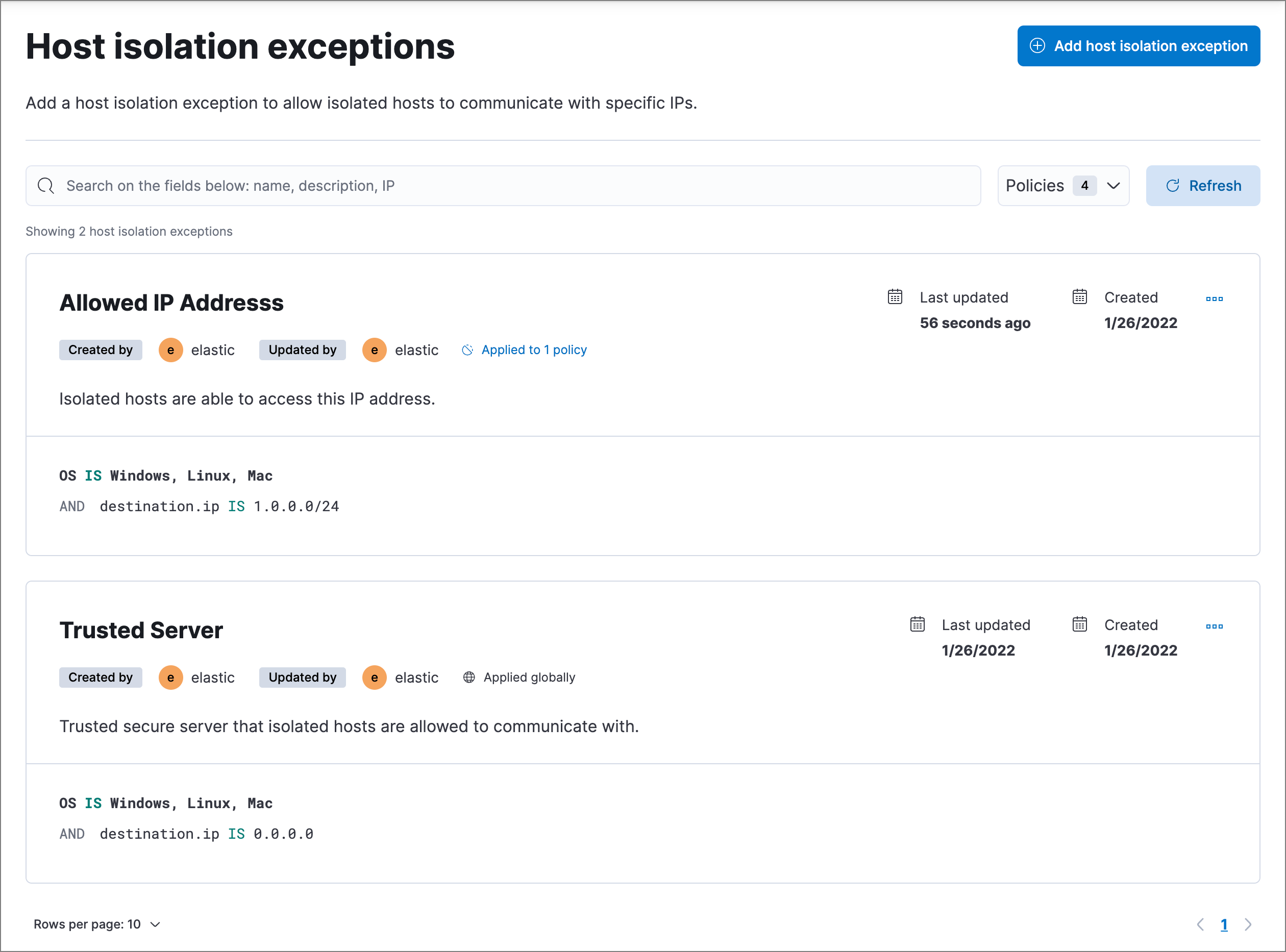The image is a screenshot of an application window displayed on a desktop computer screen. The main focus of the window is titled "Host Isolation Exceptions," prominently written in black text at the upper-left corner. Directly below this title, smaller text provides a brief description: "Add a host isolation exception to allow isolated hosts to communicate with specific IPs."

In the upper-right corner of the image, there is a prominent blue button labeled "Add Host Isolation Exception" in white text, signaling a pivotal action within this interface. Directly below this button is a horizontal search bar designed for filtering existing entries. To the right of the search bar is a drop-down box displaying the word "Policies" with the number four indicating the current selection. Adjacent to this drop-down, there is a gray refresh button with the word "Refresh" written in blue, suggesting an option to update the displayed data.

The lower portion of the window is divided into two frames. The first frame is headlined by the text "Allowed IP Addresses" in black, indicating a section where specific IP addresses that are permitted exceptions to the host isolation can be listed or managed.